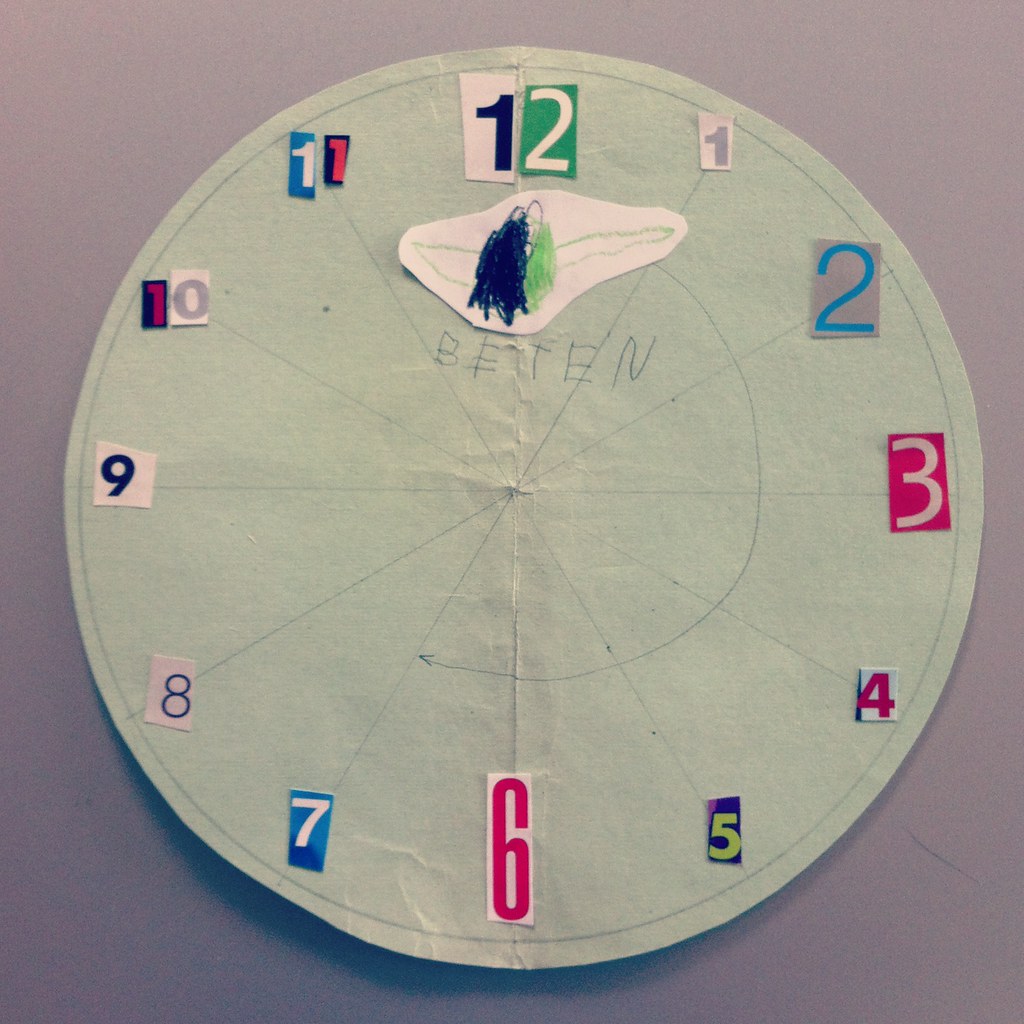This vibrant, color image features an intricately crafted clock face constructed from paper with numbers meticulously cut out from various magazines. The circular clock face, adorned in a soft, pale green hue, serves as the central canvas. From the very heart of this round shape, precise, straight lines radiate outward, seemingly drawn with a sharp pencil or pen, adding a mechanical elegance to the design. Encircling the edges of the clock face are numerals, each showcasing a unique font and a spectrum of colors, suggesting they have been sourced from diverse magazine pages. Adding a dynamic element to the composition, a curved arrow extends halfway around the clock in a clockwise direction, subtly illustrating the movement of clock hands and the passage of time.